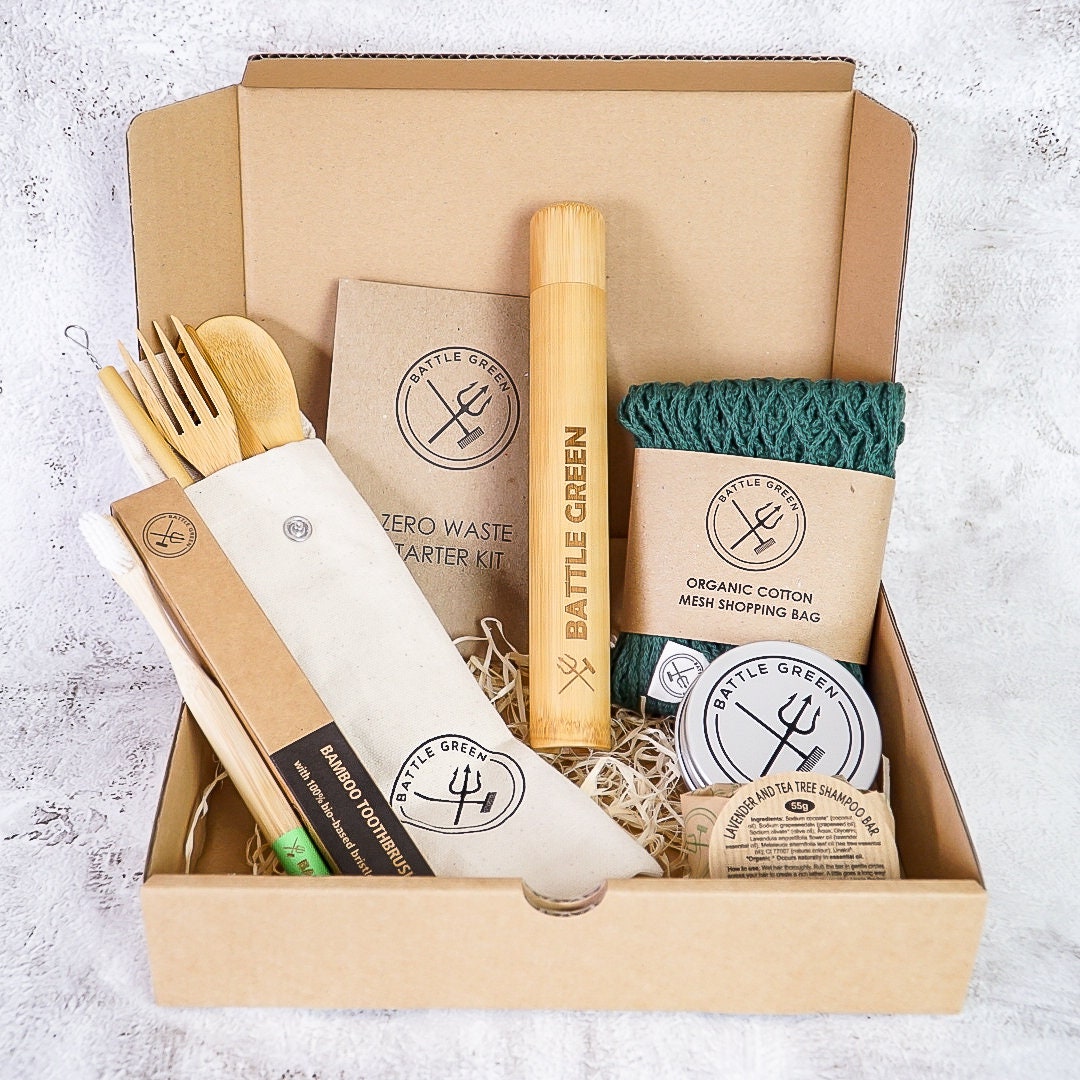The image depicts a small, tan flip-top cardboard box, sitting on a marble countertop, containing a meticulously arranged Zero Waste Starter Kit. The box is propped open, revealing a pale, grass-like filler that cradles several eco-friendly items. Prominently featured is a coiled green organic cotton mesh shopping bag, wrapped in paper labeled as such. The brand "Battle Green," identified by a logo of a pitchfork and hammer crossed in an X, is showcased on a small wooden plaque within the box. Accompanying the mesh bag is a bamboo toothbrush with 100% bio-based bristles, catering to environmental sustainability. Additionally, the kit includes wooden utensils—fork, spoon, knife, and chopsticks—and possibly a straw. A small notecard prominently displays the kit's name, reinforcing its commitment to zero waste and the use of recyclable materials.